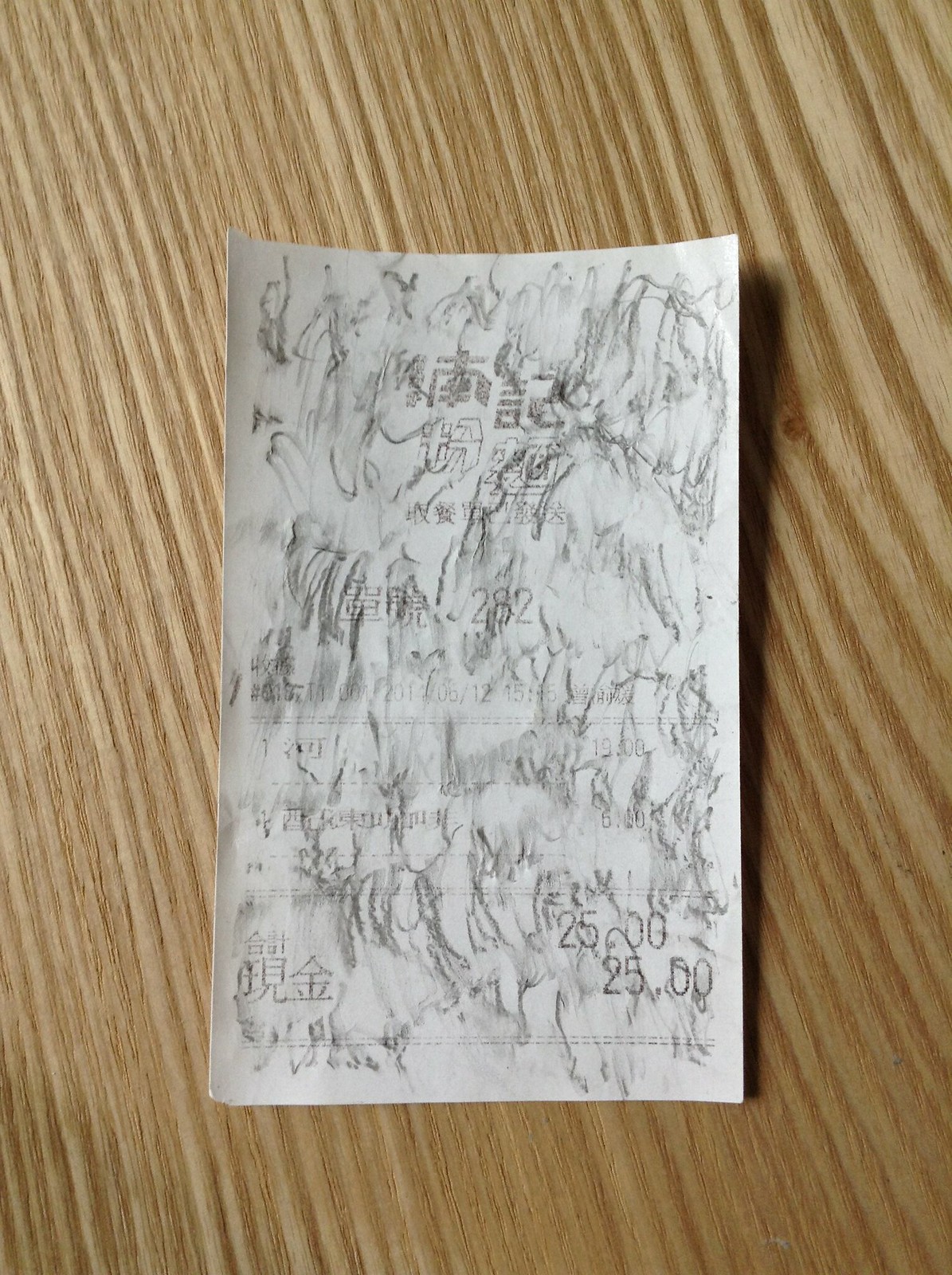A slightly curled sheet of paper, or perhaps cardboard, lies on a wooden pine table. The back of the sheet is covered in light, seemingly incoherent pencil scribbles and scrawls. Amidst the chaotic marks, a closer inspection reveals faint Asian characters, possibly Japanese, scattered across the surface. These include discernible numbers such as "282" near the center and "25.00" appearing twice towards the bottom right. Additionally, there are a few straight lines drawn across the page. Despite the overlay of random scribbles, the underlying Asian symbols and numbers suggest a hidden layer of meaning beneath the chaos.